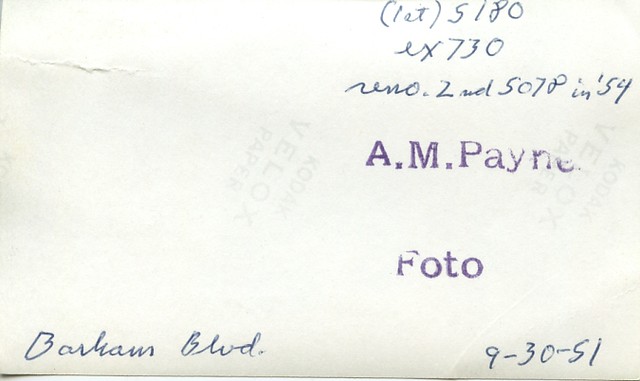This is a detailed photograph of what appears to be the back of a rectangular photo print. The paper has a few creases and features both handwriting and printed text. At the top right corner, there are three lines of handwritten letters and numbers, starting with what looks like "RET 5180" and "EX 730." Below this, it says "Reno 2nd 5078 in '54." In the center, printed in purple ink, it reads "A. M. Payne" followed by "photo," spelled as "F-O-T-O." The lower left corner has "Barham Boulevard" written in cursive script, and the lower right corner shows the date "9-30-51," signifying September 30, 1951. In the faint gray background, the paper is marked with "Kodak VELOX" and the word "paper."